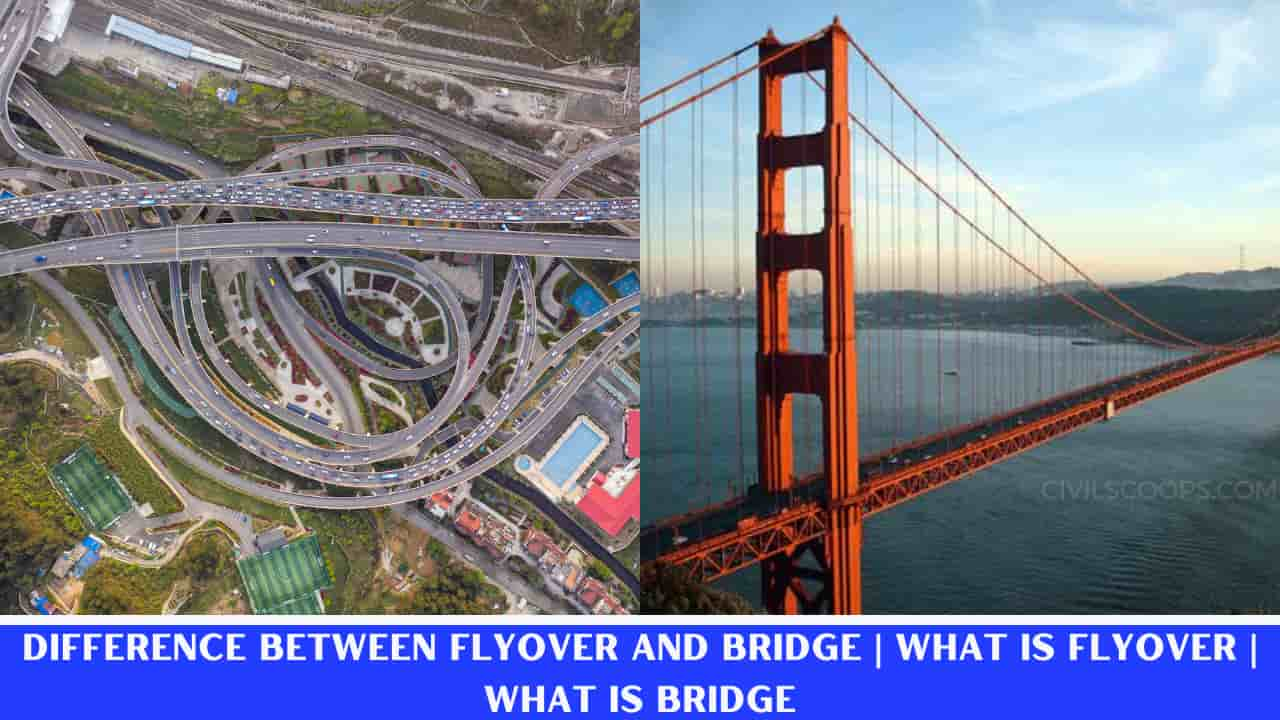The image is a comparison graphic that explains the difference between a flyover and a bridge, as indicated by the white text set against a bright blue background at the bottom of the image, reading "Difference between flyover and bridge. What is a flyover? What is a bridge?" On the left side, the image displays an extreme aerial view of a complex roadway system with multiple circular lanes, ramps, and overpasses, depicting a flyover. This view, similar to something seen on Google Maps, shows the top lane congested with cars while the bottom lane is sparsely populated. In the bottom corner of this section, some tennis courts and a swimming pool are visible. On the right side, the image features a photo of the iconic Golden Gate Bridge, an orange suspension bridge spanning the San Francisco Bay. This well-recognized structure is shown at sunset, with the golden light reflecting off its beams.